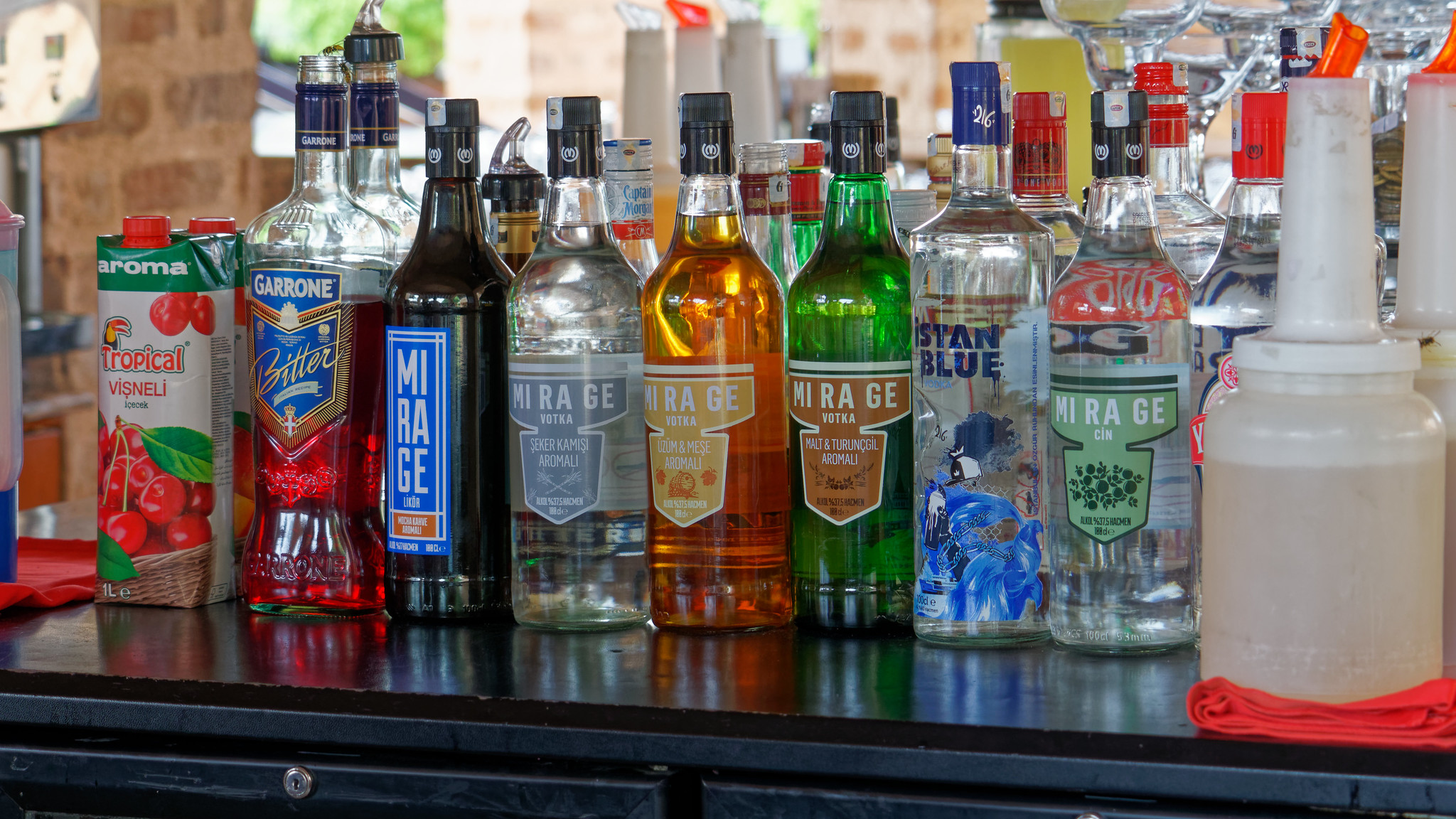The image depicts a bar setup on a black counter, featuring an array of around 30 assorted alcoholic beverages and related accessories illuminated by daylight. Most bottles prominently display the brand name "Mirage," often with the letters spaced vertically, and contain various types of clear and brown liquors. To the left, there’s a distinctive one-liter carton labeled "Tropical Visnelli," adorned with cherries and a toucan, suggesting a cherry-flavored drink. A smaller bottle with a green top and red cap, also labeled "Tropical Visnelli," sits nearby. The brand "Garone," in a black shield label, is inscribed on another bottle filled with a red substance labeled "Bitter." The bottles' vibrant colors and diverse labels stand out, adding visual interest. The setup includes elements typically found in a bar, such as cocktail shakers and glasses, which are positioned behind the bottles. The upper part of the counter features a keyhole, possibly indicating a lockable storage area. This scene captures the organized yet eclectic nature of a home bar or a small commercial bar area.